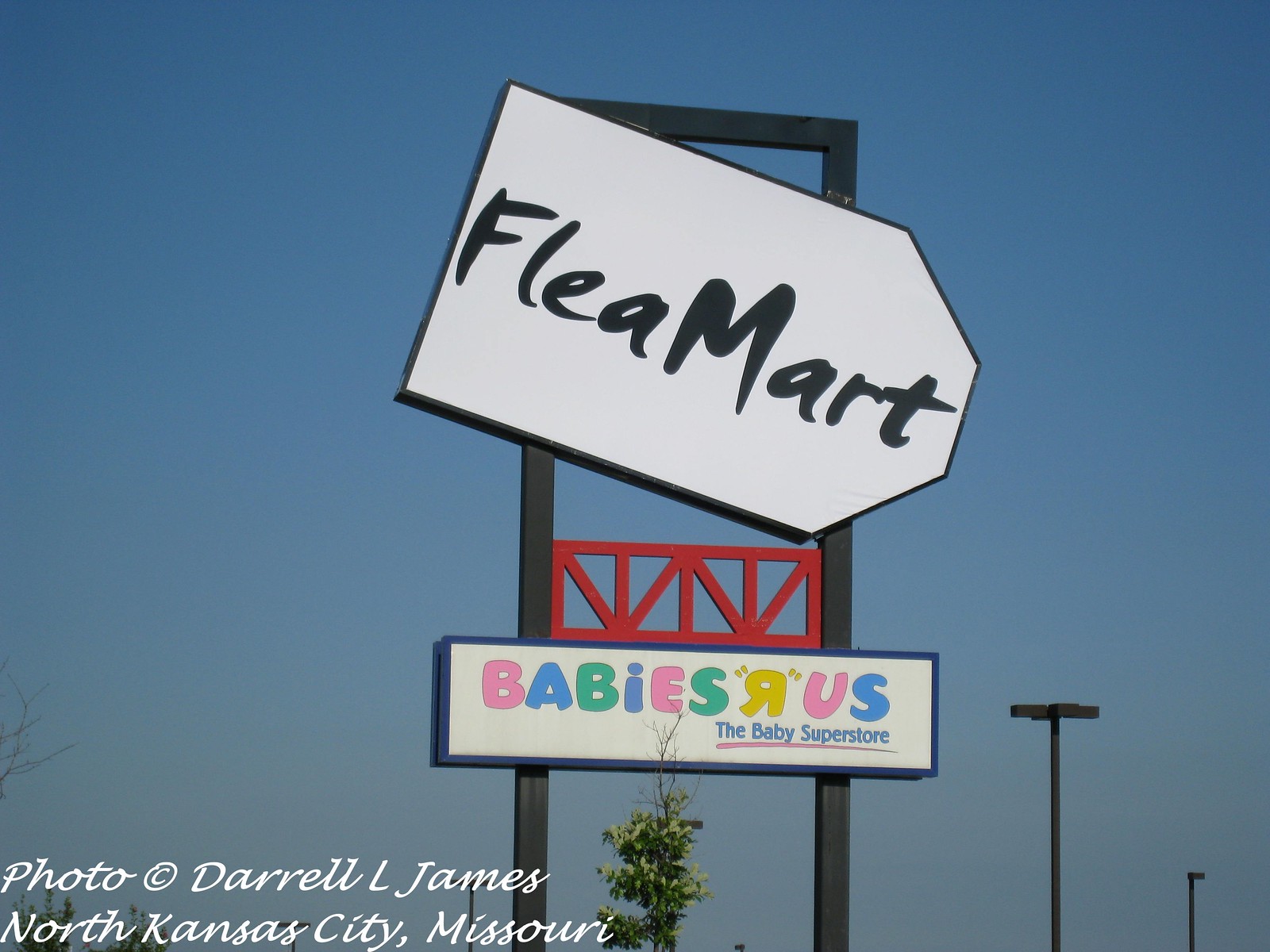The image showcases a tall shop sign set against a clear sky, appearing to be situated in a parking lot, though the ground and surrounding areas are not visible. The primary sign is supported by two tall metal struts and features a white background with bold black text reading "Flea Mart." The design of the sign mimics the familiar outline of a Best Buy tag. Beneath the Flea Mart sign is another sign, labeled "Babies R Us," accompanied by the tagline "The Baby Superstore." This secondary sign displays a white background adorned with colorful text in shades of pink, blue, and green. In the bottom left corner of the image, the text "Photo Copyright Darryl L. James, North Kansas City, Missouri" is visible.